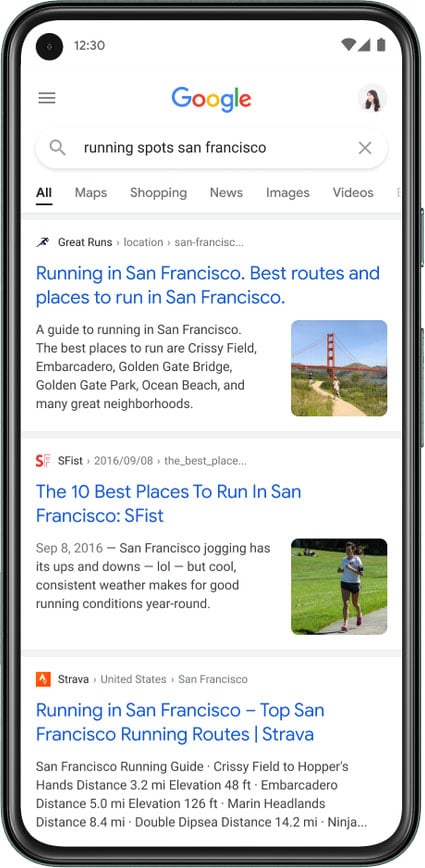**Descriptive Caption for Screenshot of Smartphone Displaying Running Routes in San Francisco**

The image captures a smartphone screenshot, showcasing the silver outline of the phone set against a white background. At the very top left corner, a black circle indicates the time, displayed as "12:30". On the top right corner, the icons for Wi-Fi reception, phone signal strength, and battery status are visible.

Centrally positioned at the top, the familiar multicolored Google logo (blue, red, yellow, and green) is prominently displayed. Directly below the logo, a search text box contains the query, "Running Spot San Francisco."

Beneath the search box, navigation tabs are lined up horizontally: All, Maps, Shopping, News, Images, and Videos. Three detailed entries about running in San Francisco follow:

1. **First Entry:**
   - **Header:** Great Runs
   - **Click Title:** Running in San Francisco, Best Route and Places to Run in San Francisco.
   - **Description:** The Best Guide to Running in San Francisco. The Best Places to Run are Crissy Field, Muir Woods National Monument, Golden Gate Bridge, Golden Gate Park, Ocean Beach, and many great neighborhoods.
   - **Image:** An iconic picture of the Golden Gate Bridge.

2. **Second Entry:**
   - **Title:** The 10 Best Places to Run in San Francisco
   - **Date:** September 8, 2016
   - **Description:** "San Francisco Jogging has its ups and downs, LOL, but cool consistent weather makes for good running conditions year round."
   - **Image:** A runner jogging next to a lush green field.

3. **Third Entry:** (Strava Selection)
   - **Title:** Running in San Francisco, Top San Francisco Running Route
   - **Source:** Strava, United States, San Francisco
   - **Instructions:** 
     - **Crissy Field to Hopper’s Hands:** Distance: 3.2 miles, Elevation: 48 feet
     - **Muir Woods to Sierra Road:** Distance: 5 miles, Elevation: 126 feet
     - **Marin Headlands:** Distance: 8.4 miles
     - **Double Dipsea:** Distance: 14.2 miles, Ninja

This screenshot provides comprehensive information and images that guide users through the best running routes in San Francisco.